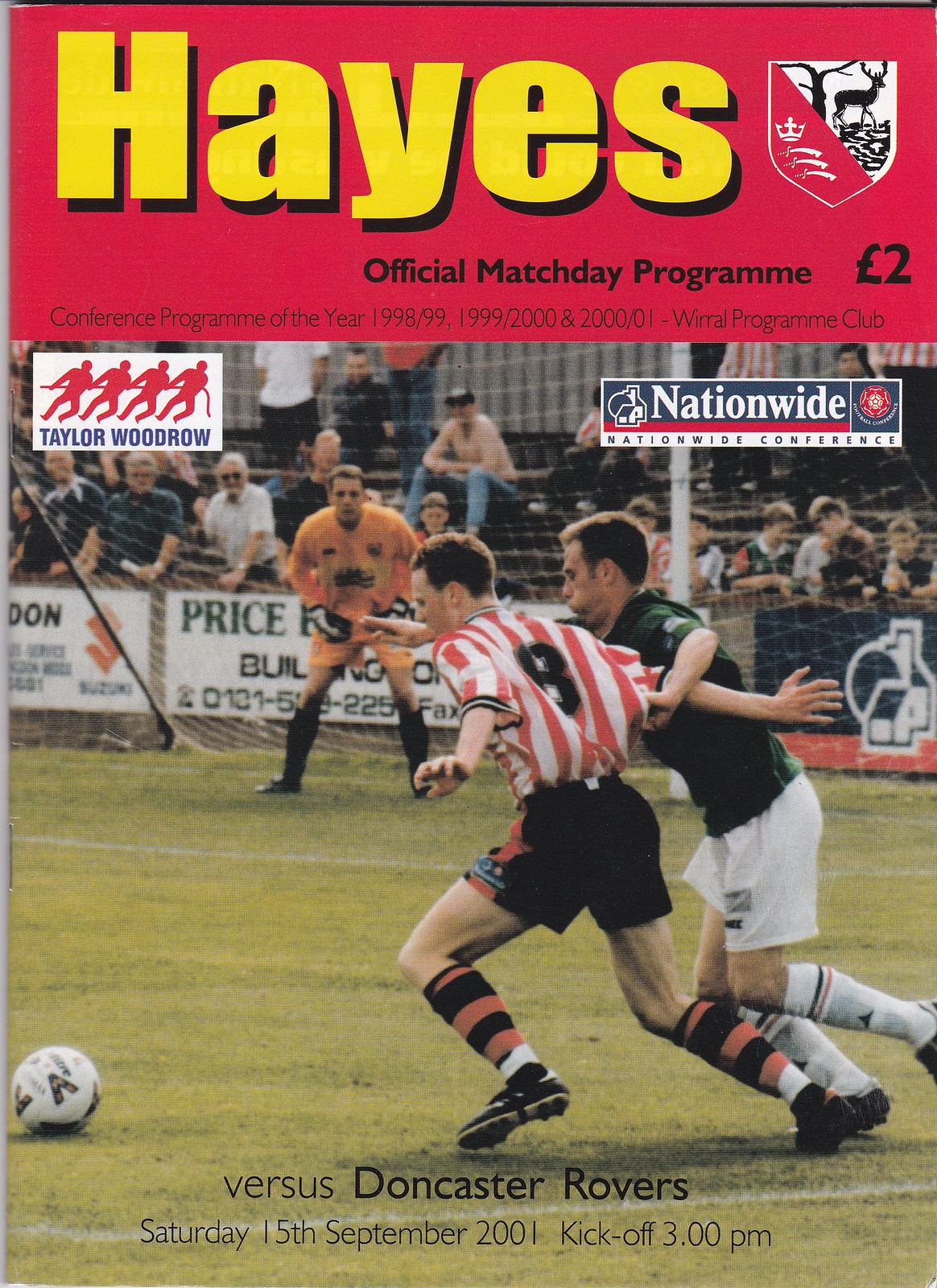The image depicts a detailed program brochure for a sporting event, specifically a soccer match. The top third of the image has a red background, featuring the word "Haze" in a large yellow font with black detailing on the left-hand side. Adjacent to the text is a divided crest; the bottom half of the crest has a red background with a white crown, while the top half features a black tree and deer on a white background. Beneath the main heading and logo, in black font, it reads "Official Match Day Program," priced at two pounds. Following this, another line states, "Conference Program of the Year 1998/99, 1999/2000, and 2000/01 - World Program Club."

The bottom two-thirds of the image shows an action-packed photograph from a soccer game. In the background, a goalie, wearing an orange jersey, shorts, black cleats, black socks, and black-and-white gloves, stands near the net. He is a Caucasian male with short brunette hair. In the foreground, two soccer players are competing for the ball positioned at the bottom left of the frame. The player in the middle of the image, also Caucasian with short brunette hair, is dressed in a vertically striped orange and white jersey with the number eight in black on the back, black shorts with orange detailing, horizontally striped orange and black socks, and black cleats. To his right, another Caucasian player with short brown hair is seen wearing a deep green jersey, white shorts, white socks, and white cleats.

At the very bottom of the photograph, in black font, the text reads "versus Doncaster Rovers, Saturday 15th September 2001, kickoff 3 p.m." Additionally, advertisements at the top of the image include a rectangular white box on the left with an image of four red stick figures pulling a rope, captioned "Taylor Woodrow" in blue font. On the right-hand side is another advertisement in navy, white, and red colors with the large white text "Nationwide."